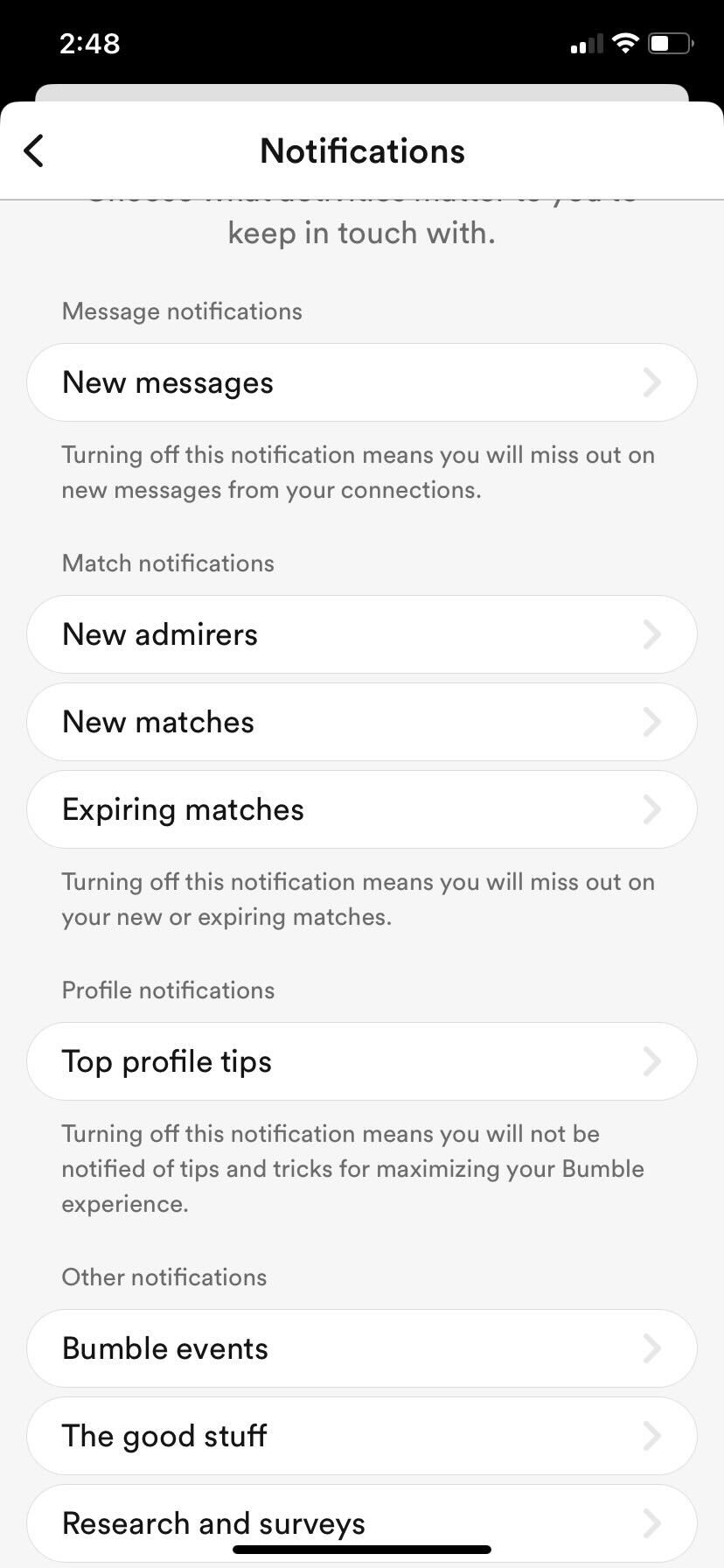**Caption:**

This detailed screenshot from a phone, captured at 2:48, highlights the notification settings page within the Bumble app. At the top, it displays headings such as "Notifications," "Message Notifications," and "New Messages." An explanatory message under "New Messages" alerts users that disabling notifications will result in missing new messages from their connections.

The settings options available include toggles for various types of match notifications: "New Admirers," "New Matches," and "Expiring Matches." Further down the page, there's a section called "Profile Notifications," featuring "Top Profile Tips" to help users enhance their profile's attractiveness.

Additional notification settings pertain to promotional content within the app, including "Bumble Events," "The Good Stuff," and "Research and Surveys." This combination of notification management and promotional information aims to improve user experience and engagement on the Bumble platform.